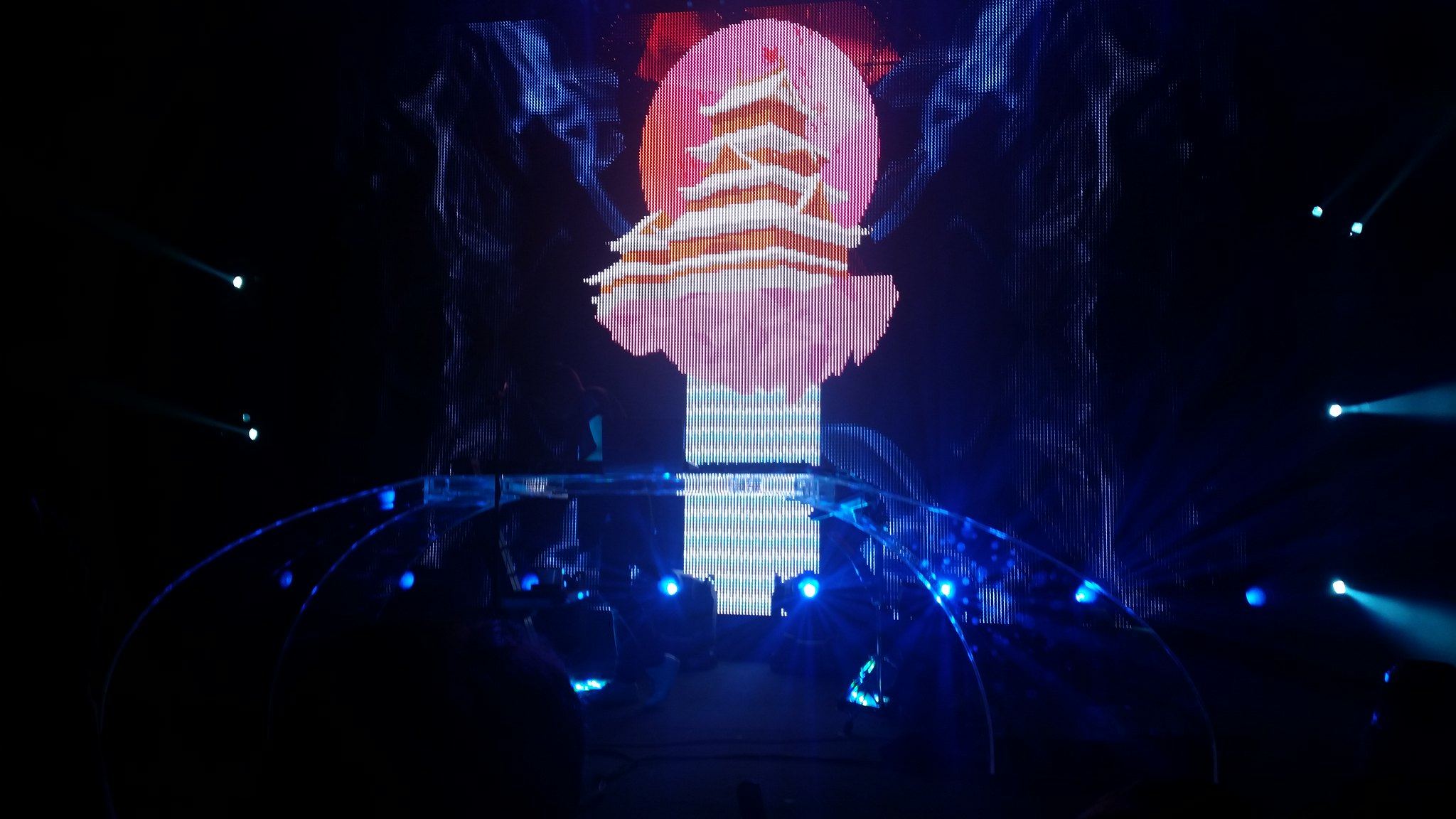The image captures a mesmerizing indoor holographic show in a dark, blackened environment. At the center is a stunning projection of a multi-tiered pagoda or temple. This structure boasts brownish wood-colored walls adorned with white, snow-like roofs on each layer. The temple is elevated, seemingly floating above a collection of delicately pointed, downward-facing pink rocks or a floating pink ground.

A large, luminous pink circle resembling a sun serves as a backdrop to the temple, enhancing its ethereal appearance. Projected lights, some bluish, are shining upwards from the bottom, creating a light haze of fog or smoke that adds a sense of mystique and depth. The setup is surrounded by multiple light sources and smaller screens, framed and supported by beams curving towards the central display. Below and behind the structure, there appears to be a blue, possibly fantastical element resembling a skyscraper or a waterfall, enhancing the otherworldly ambiance of this captivating holographic presentation.